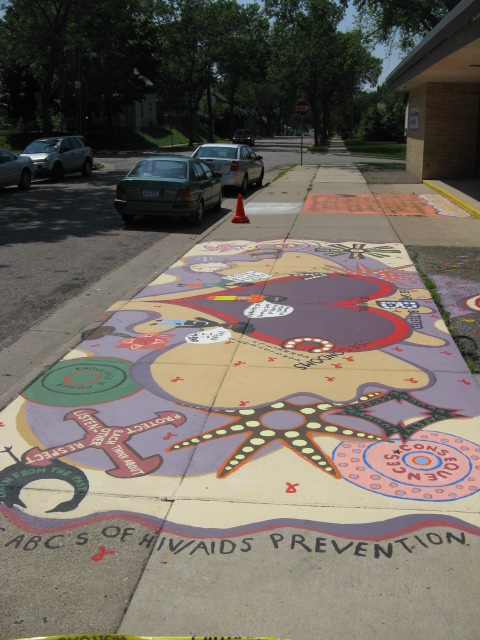The photograph captures a lengthy, colorful sidewalk mural dedicated to the ABCs of HIV/AIDS prevention, extending across several sidewalk squares in a vibrant display of artistry. This mural, composed of either chalk or paint, spans from the street toward an undefined building, possibly a school or picnic shelter. The mural showcases a collage of various shapes and symbols including a prominent purple heart outlined in red, a starfish, a red cross, and a pink ball with blue circles, with words like "Consequences" interspersed throughout. The sidewalk is flanked by parked cars, some on either side of the adjacent street, with a lone traffic cone situated on the sidewalk. The scene is framed by residential housing on the left and a brick building on the right, under the canopy of background trees, creating a tunnel-like perspective that draws the viewer into the intricate and meaningful artwork.